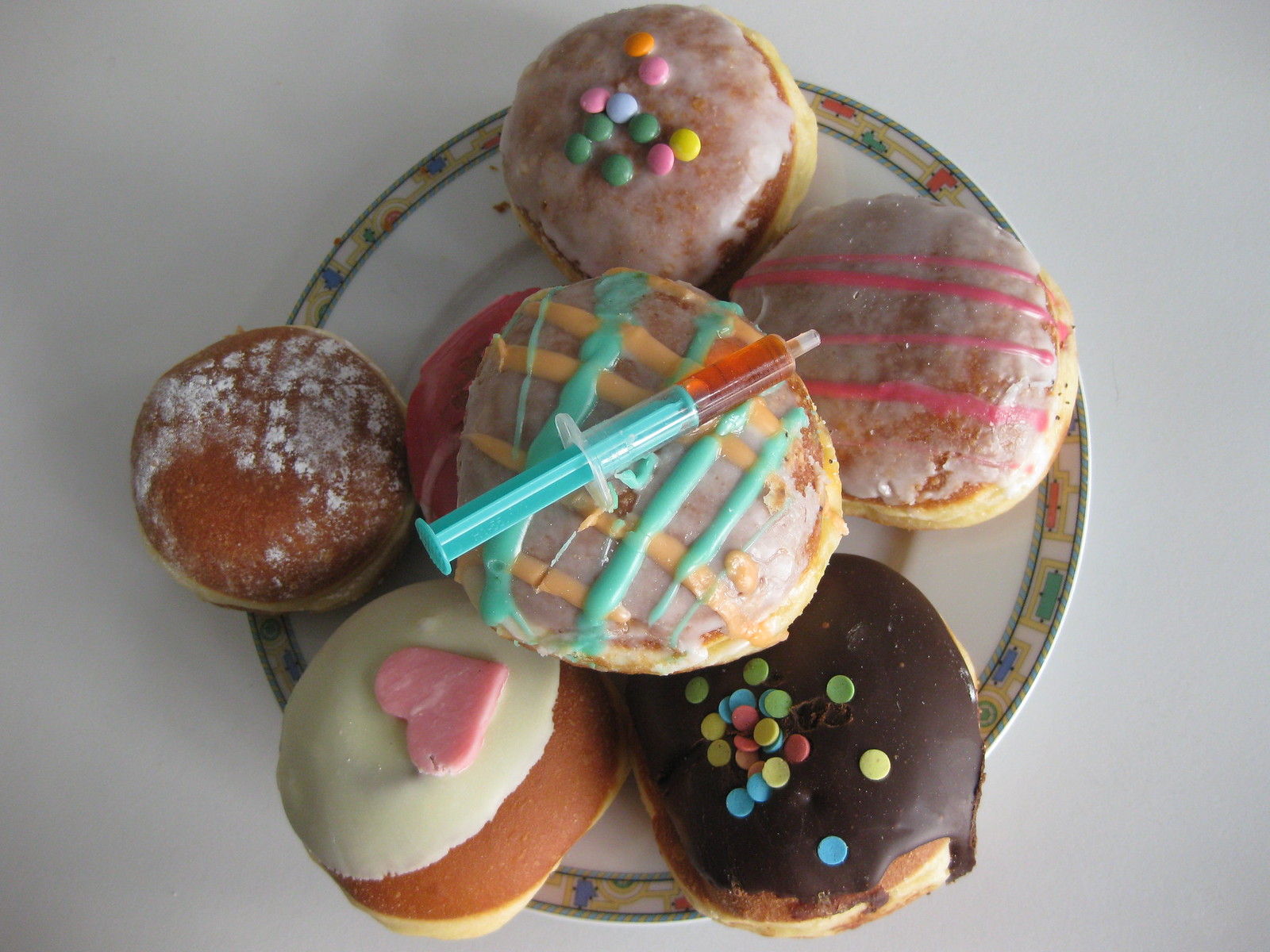In the image, a white plate with an intricate border composed of yellow squares with blue, green, and orange accents is set against a light orchid background. Arranged in a circular pattern, the plate holds six distinctively decorated donuts, with one prominently placed at the center. Starting clockwise from the top, the first donut is cream-filled, adorned with white frosting and a heart-shaped decoration. Next is a chocolate-filled donut coated with chocolate frosting and speckled with circular sprinkles in blue, yellow, and pink, along with hints of green. Moving on, there's a donut with white frosting, crisscrossed by pink stripes, another with similar white frosting capped with what appear to be light-colored Skittles or M&M's. The fifth donut on the far left is lightly frosted and semi-cream-filled. The central donut stands out with its unique topping: white frosting beneath which lies a pink layer, enhanced with yellow and blue streaks, crowned by a syringe filled with a brownish liquid. Each donut is meticulously designed, adding vibrant variety to the ensemble.